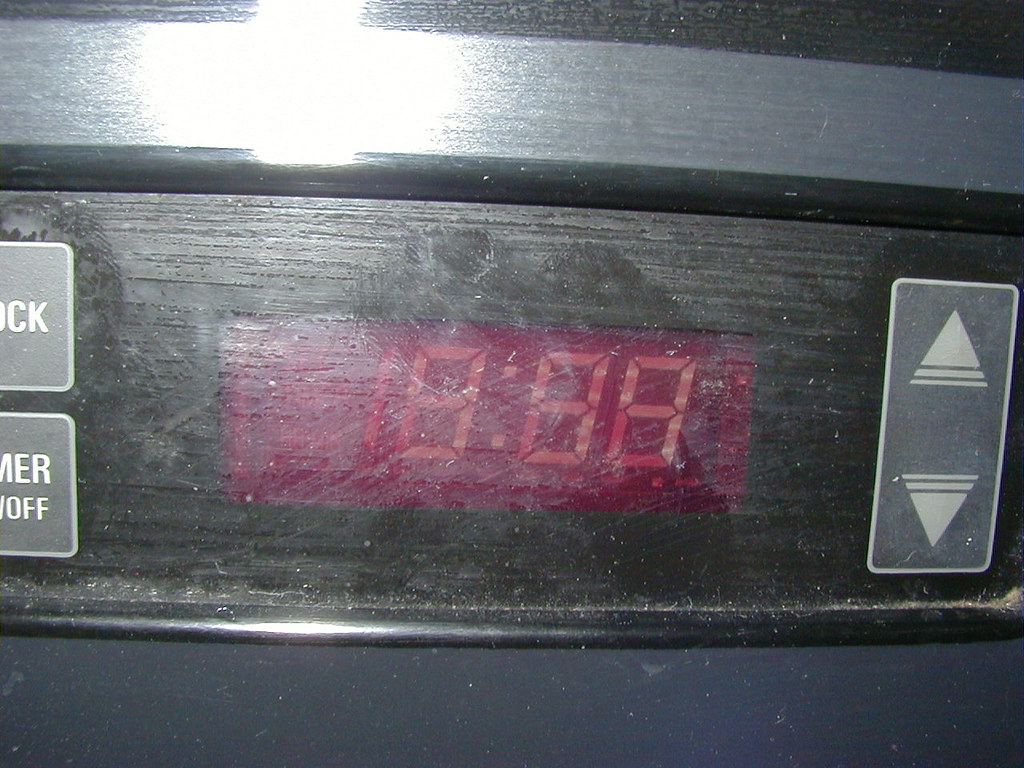This is a close-up, zoomed-in view of a stove or oven clock set against a background of brushed silver metal. The clock, a large black rectangle with a thin black border, features a central digital display with red numbers. To the left of the digital face, there are two vertically aligned gray buttons with white outlines and letters: the top button labeled "Clock" and the bottom one labeled "Timer On/Off." To the right, there is a large vertical rectangle with an "Up" and "Down" triangle for adjustments. The display face shows signs of wear, with fingerprints and dust collected in the corners. Additionally, there is noticeable dust buildup in the right corner and along the bottom edge, accompanied by smears and fingerprints on the front surface, giving it a dirty appearance.